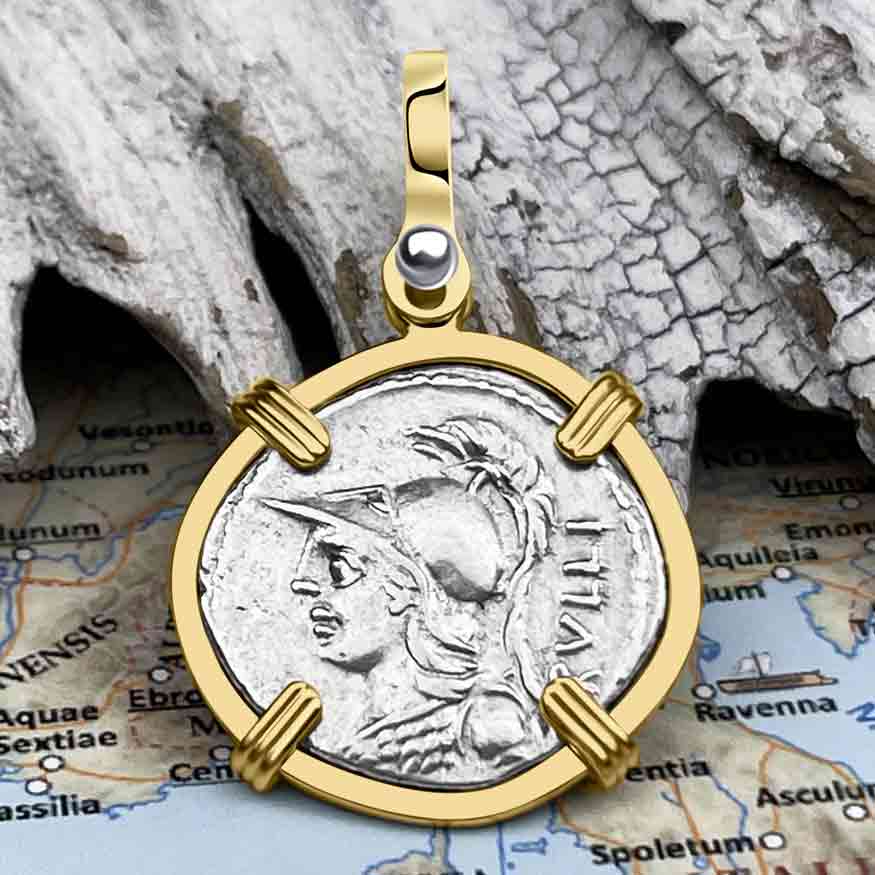This image features a roughly quarter-sized, silver coin, prominently displaying the profile of a Roman soldier adorned with a detailed helmet, complete with a visor and plume feathers. The soldier's face, characterized by a large nose, mouth, and eyes, looks leftward. The coin is irregular in shape with visible dents, giving it an antique appearance.

The coin is encased in a custom-made, gold-colored holder that secures it in place with four clasps—two from the bottom and two from the top—and features silver rivets. This casing is designed to be worn as a pendant, evidenced by a clasp at the top for threading a necklace.

The entire setup is propped against a piece of rugged, bark-like wood and rests upon a map. The map beneath, predominantly blue with tan land masses, appears to depict the Mediterranean region, possibly hinting at the Roman Empire's historical context. The meticulous presentation suggests the image might be intended for showcasing the coin as a collectible or a piece of jewelry for sale.